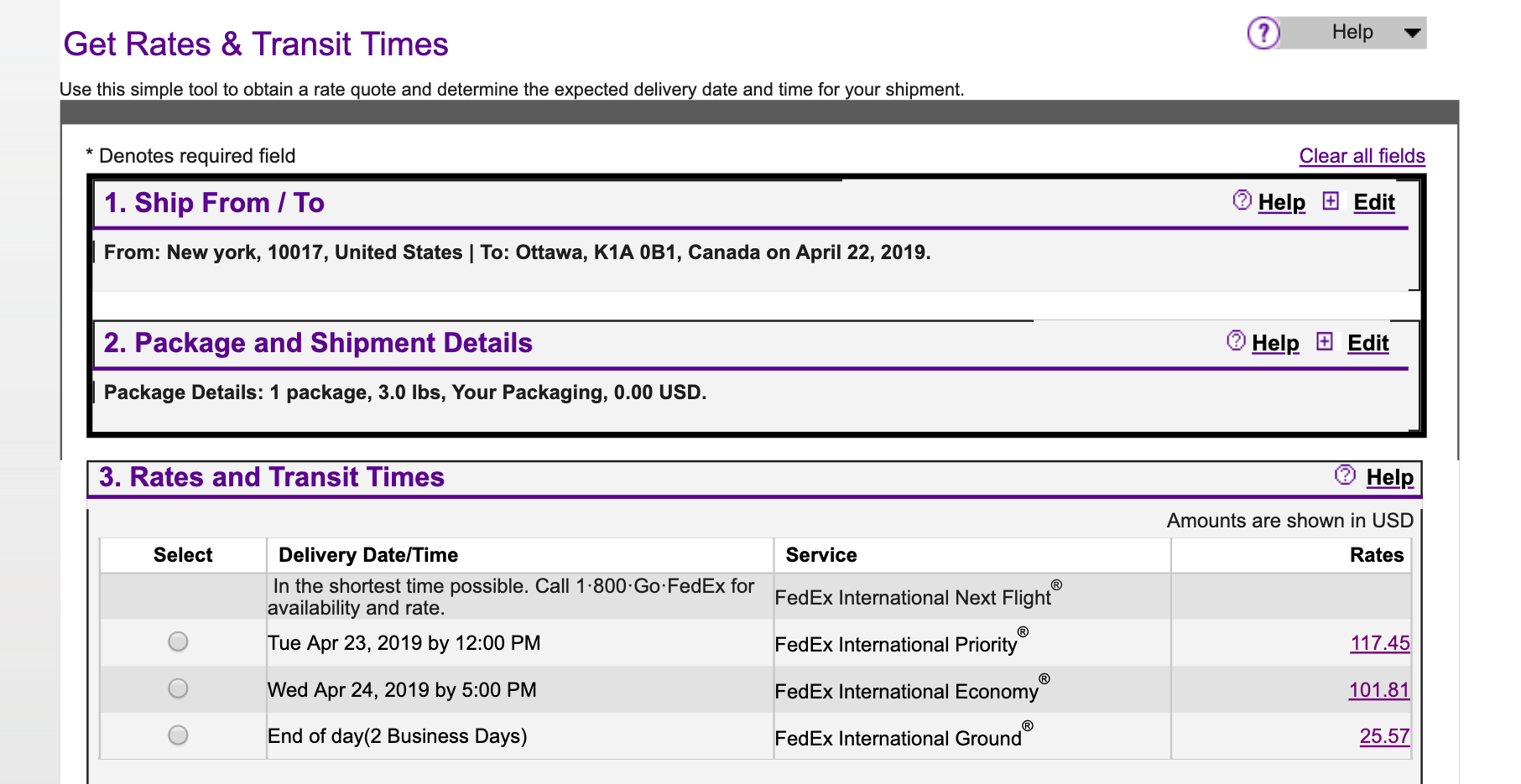Description: This website displays a detailed shipping form with various options for choosing different services, each priced differently. The form enables users to get a quote for their parcel shipment, providing an estimated delivery date and time.

1. **Shipping Information**:
    - **From**: New York, NY 10017, United States
    - **To**: Ottawa, K1A 0B1, Canada
    - **Date**: April 22, 2019

2. **Package and Shipment Details**:
    - **Number of Packages**: 1
    - **Weight**: 3 pounds
    - **Declared Value**: \$0 USD

3. **Rates and Transit Times**:
    - The form features a four-column table with three service options:
        - **Priority**
        - **Economy**
        - **Ground**

This setup allows users to select their preferred shipping method based on a comparison of the available rates and estimated delivery times.